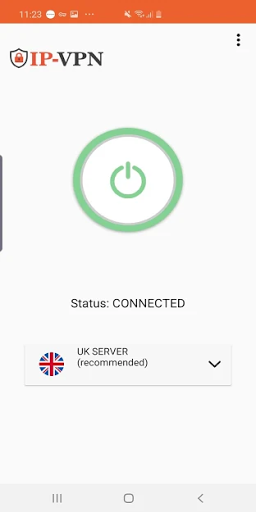The image depicts a smartphone screen in portrait mode. At the top, in a red area, the time "11:23" is displayed in white, flanked by various status symbols including a key, an image icon, a battery icon, Wi-Fi signal strength, and reception indicators. Below this, the text "IP-VPN" is prominently displayed in red, accompanied by a black outline of a shield with a red lock inside. To the right of this, three vertical black dots are arranged in a column.

Further down, a green power button is visible, characterized by a green outline, a white center, and a green circle with a line at the top. Directly below, the status "CONNECTED" is written in black uppercase letters. A dropdown field underneath reads "UK Server (Recommended)", next to which is the UK flag icon.

At the bottom of the screen, typical user interface elements are present: a square icon in the middle flanked by three horizontal lines on one side and an arrow pointing left on the other side.